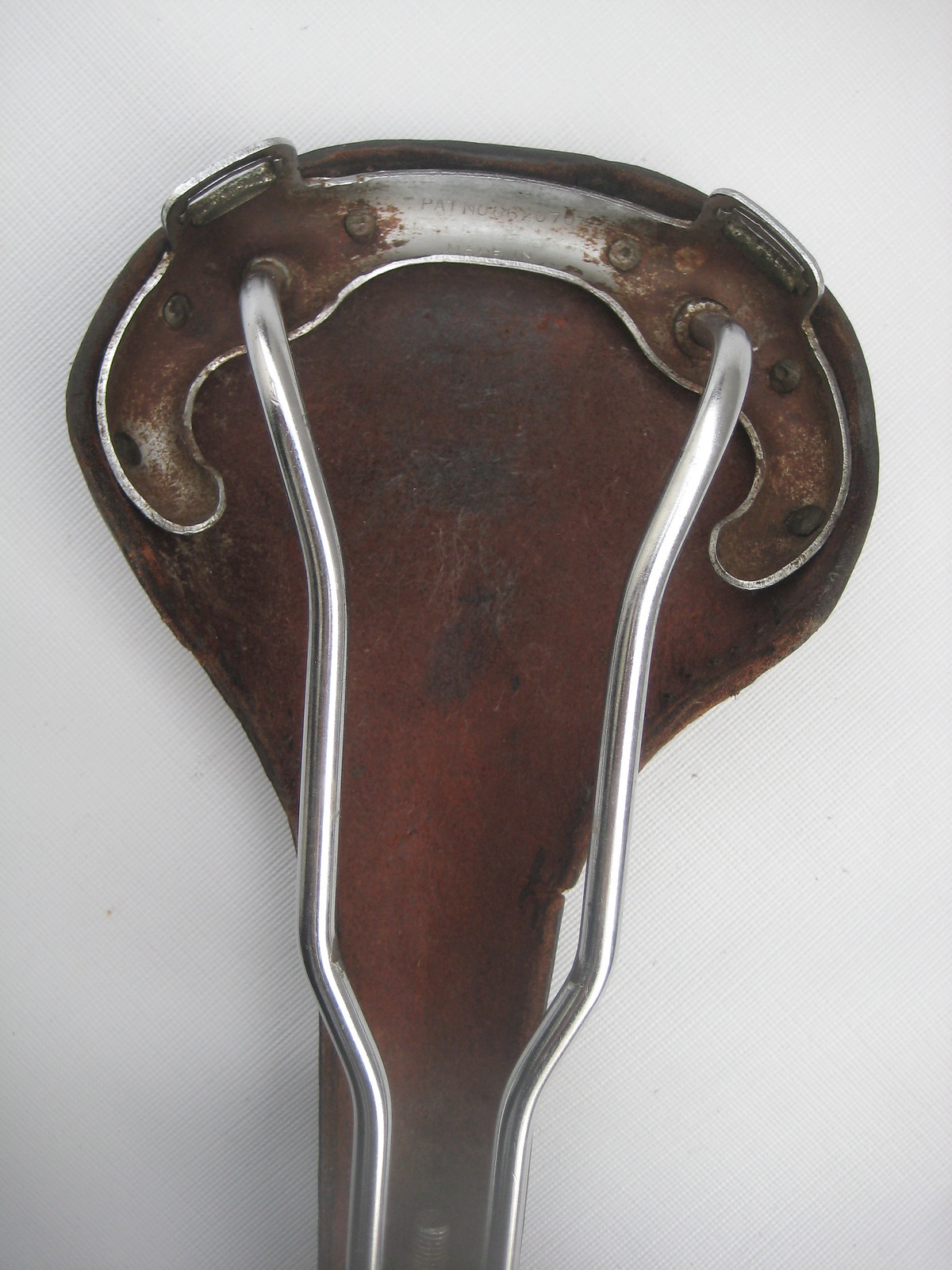The image depicts an unusual utensil-like object that is approximately five inches long. The central part of this item is brownish in color, indicating that it is either made of wood or heavily rusted metal. The shape of this central segment resembles a gumdrop or an elongated oval, wider at the top and narrowing towards the bottom. 

Attached to this central segment are two long, thin, silver metal handles or poles that run vertically along the left and right sides of the object. These silver handles appear slightly bent or curved. The top part of the object, where the handles meet, features a silver metal plate that seems integral to the design. This metal plate and the surrounding area show signs of rust, adding to the aged and weathered appearance of the item. The entire object is set against a white background for contrast. Despite its peculiar design, the exact purpose of this item remains unclear.